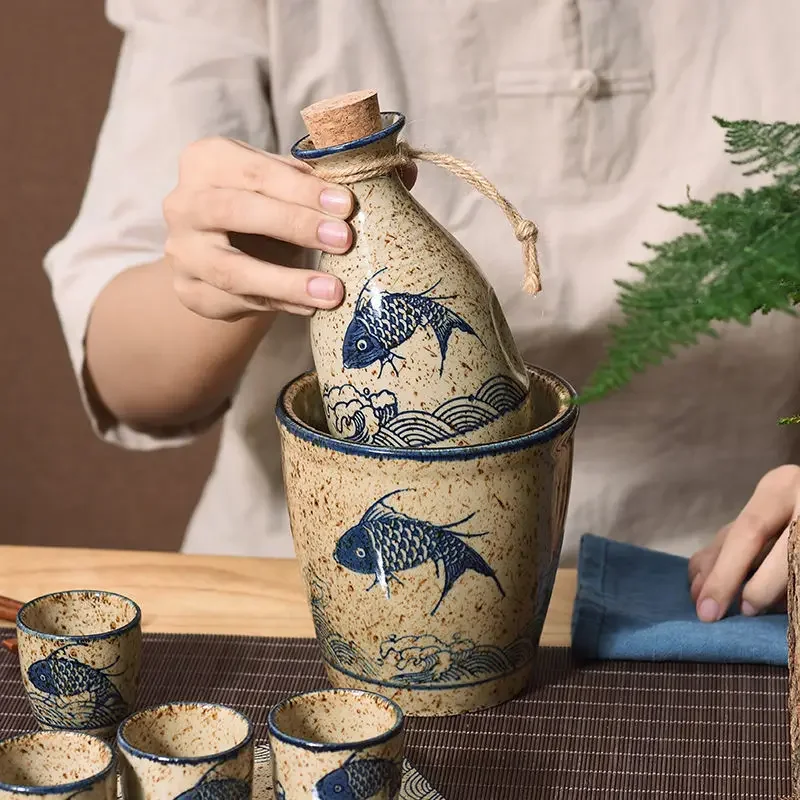In this detailed image, a person with neatly manicured hands is interacting with a set of artistically crafted ceramic pieces on a wooden table covered with a dark brown thatched mat. The centerpiece is an old-style tan ceramic bottle with a cork stopper and a piece of twine wrapped around its neck, featuring a stylized koi fish and wave patterns in blue. The bottle, with dark brown speckles and a sandstone hue, is being pulled from a matching ceramic bowl by the person's right hand. Only part of the person's torso is visible, clad in a shirt with an ambiguous pocket or fastener. Their left hand presses down on a blue dishcloth. In the foreground, aligned on the left, are four smaller shot glass-like cups, each adorned with the same koi fish and wave motif. Adding a touch of nature, a green fern branch enters the frame from the right. The scene has a photorealistic quality, suggesting careful artistic intent or AI generation.